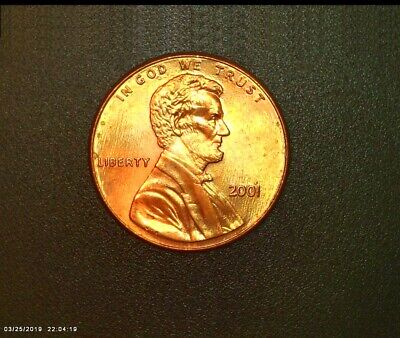This image showcases a detailed depiction of a 2001 Lincoln head penny, a piece of American currency worth one cent. Positioned on a dark grayish-black surface, the copper penny gleams under a direct light source. The penny prominently features the iconic side profile of Abraham Lincoln facing right. Lincoln, known for being president during the Civil War, is depicted in a formal jacket with a bowtie and his neatly trimmed hair and signature beard. Engraved above his head are the words "In God We Trust," while "Liberty" is inscribed to his left and the year "2001" to his right. On the bottom left corner of the image, a date stamp reads "03/25/2019" and "220419" in small white lettering. This penny, a familiar fixture in American numismatics, continues to be a significant emblem of the nation's history and currency.